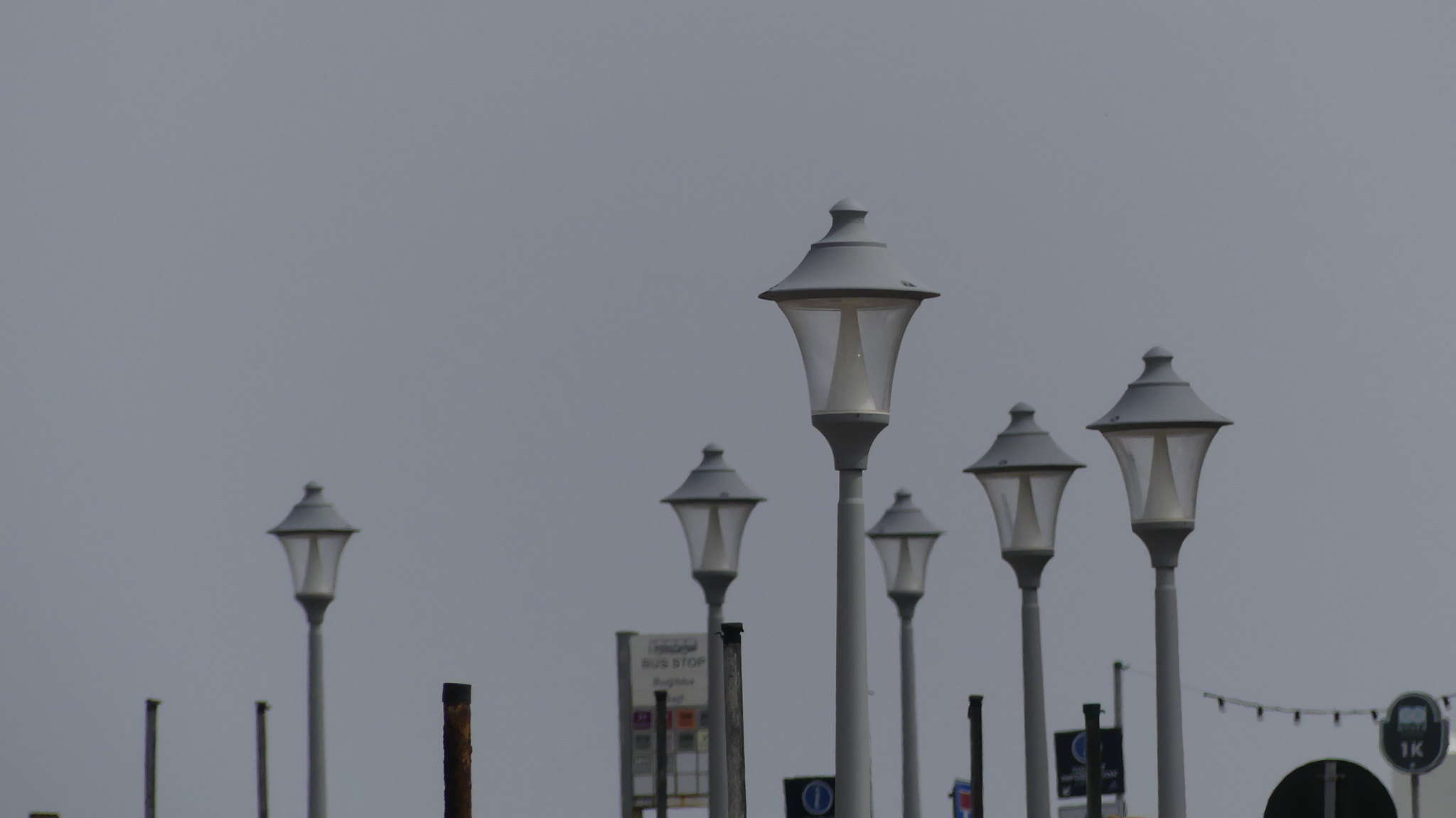This photograph captures a cloudy, overcast day, presenting an array of six identical street lamps arranged along a park or perhaps a pier-like area. These lamps, constructed from light gray metal, feature a unique design with triangular tops that flare outward, leading down to a glass section that tapers inwards, resembling an inverted cone housing the bulb. While the sky remains uniformly gray, the daylight is subdued, filtering through thick clouds, suggesting a lack of direct sunlight but no indication of rain. The lamps are arrayed in an interesting pattern: the three on the right are closely bunched together, while the three on the left are more spaced out, with the middle left lamp being the nearest. The base of these lampposts is not visible in the image, hinting at varying heights in the photo’s perspective. In the backdrop, there are additional poles without any lamps, adding to the industrial ambiance. Prominently, there’s a bus stop sign, rectangular in shape with some smaller colored squares beneath it, positioned slightly in the background, approximately ten feet from the nearest street lamp. This sign, along with others that are unreadable, subtly confirms the location as likely being a public transit area, enhancing the urban feel of the scene.